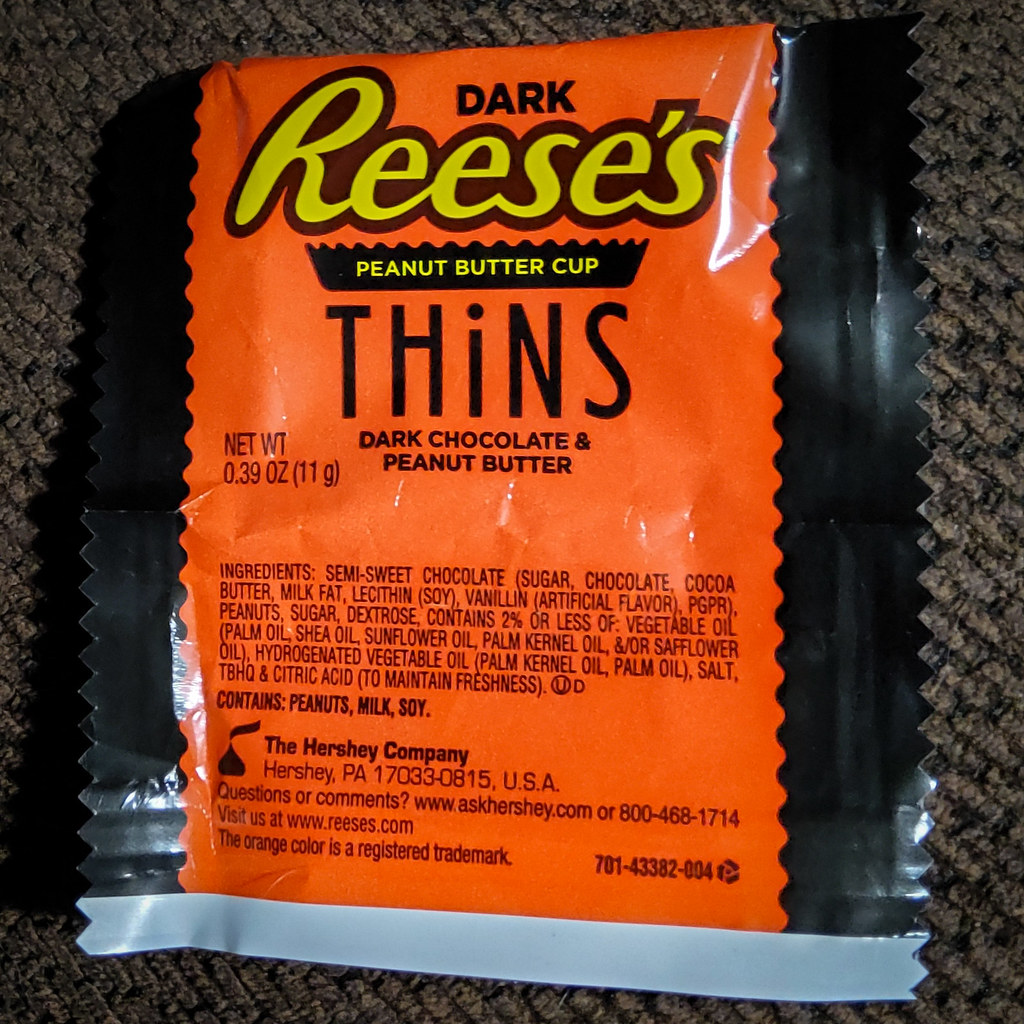This photograph showcases a package of Dark Reese's Peanut Butter Cup Thins. The wrapper predominantly features an orange color scheme with brown accents on the sides and a silver stripe along the bottom edge. The text on the packaging is remarkably clear and legible, including the fine print. The word "Dark" appears in smaller lettering, while "Reese's" is prominently displayed in bold yellow lettering. Below it, "Peanut Butter Cups" is written in smaller yellow letters against a backdrop illustration of a peanut butter cup. The word "Thins" is prominently bold in larger brown letters. Further details include the phrase "Dark Chocolate and Peanut Butter" in small brown letters.

The net weight is specified as 0.39 ounces (11 grams). The packaging also lists all the ingredients, followed by bold allergy information stating the product contains peanuts, milk, and soy. The manufacturer's details are noted as The Hershey Company, located in Hershey, Pennsylvania, accompanied by the Hershey's Kiss symbol and a trademark indication. Lastly, a small recycling symbol is present in the bottom right corner, suggesting that the wrapper is recyclable.